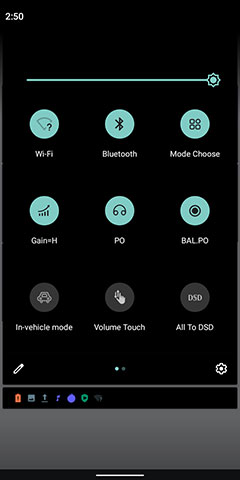The image displays a user interface on a black background with several elements visible. A large "250" is prominently featured in the background, surrounded by elements highlighted by full sunlight. In the interface, the Wi-Fi and Bluetooth toggles are enabled, while the gain setting is marked as "H." The label "PL" is visible, likely signifying playback or playlist.

A bar indicating the status of the vehicle mode is not toggled, suggesting the device remains in standard operation mode. The volume control is set to DSD (Direct Stream Digital), indicating high-resolution audio playback. The battery icon is visible, alongside various symbols including a photo, music note, blue circle, gray shield, and gray rectangle, though their specific meanings are unclear.

Additionally, a white line and a black bar are part of the interface elements. The overall theme of the display utilizes a black background for contrast and clarity.